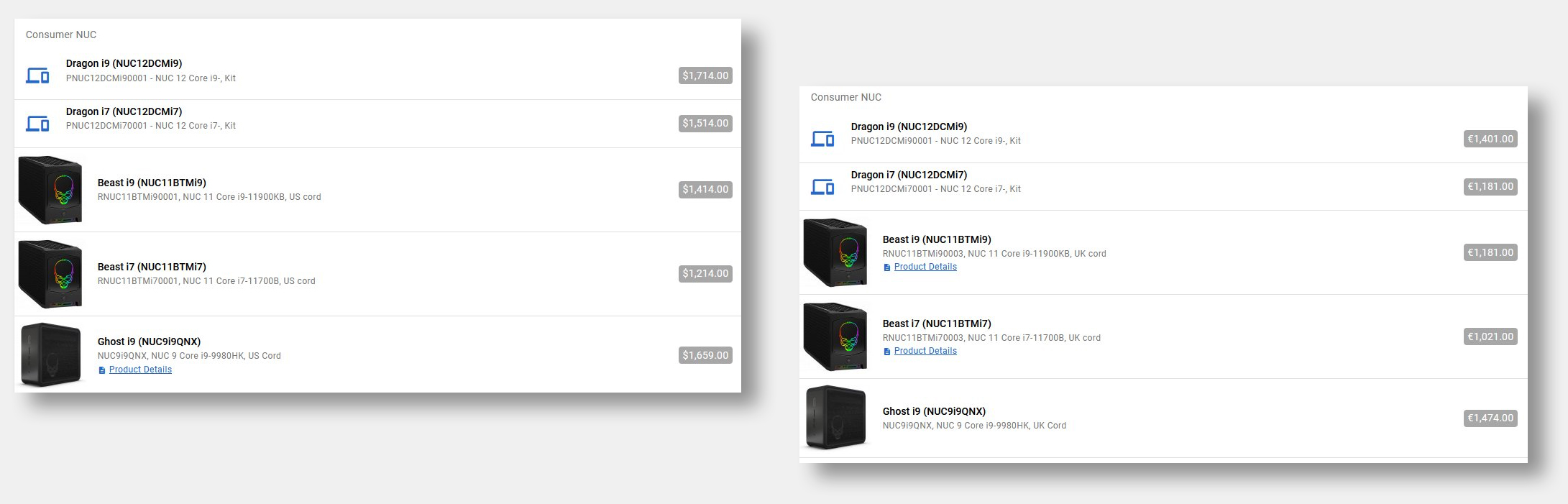Caption: 

"The website features two distinct, yet similar, web pages with a predominantly gray background and white content boxes at the center. Each webpage contains five divided sections adorned with both text and images. In the first webpage, the sections include small black text at the top, two computer-generated blue images, and three large black boxes that possibly contain images relevant to the accompanying text. The second webpage mirrors the first in structure but with slight variations: it too has two blue images accompanied by black text, while the remaining three boxes are black with additional green and pink highlights. A unique gray sidebar appears on both pages, possibly indicating dollar amounts or other numerical data. Although visually organized, the text is notably small and challenging to read. The upper left-hand corner features an indistinguishable element that could be either text or numbers. Despite its clarity in layout, improved font size for readability is recommended."